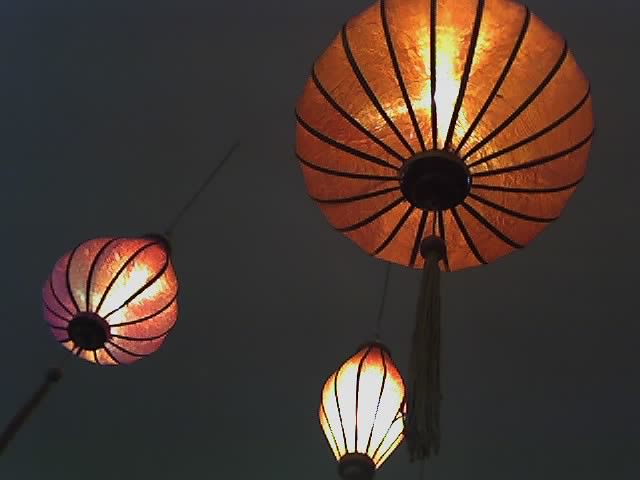The image captures a serene nighttime scene featuring three hanging lanterns suspended against a dark, nearly black background, which could either be an outdoor night sky or a very dimly lit indoor ceiling. The perspective is from below, looking up at the lanterns, which appear to be floating due to the darkness surrounding them. 

The lantern in the bottom left corner is attached to a slender black pole with a circular base, extending upwards. This lantern has an oval shape tapering to a point at the top, with a soft red glass segmented by evenly spaced black lines and crowned with another black base from which a chain hangs. The second lantern, positioned towards the center of the image, is narrower and almost diamond-shaped, exhibiting a bright, almost white hue with red tinges at the top. The third lantern, just right of center, is rounder and more circular, glowing with an orange light and also segmented by black lines.

All three lanterns share a design featuring vertical black lines and long tassels hanging from their bases, adding a traditional touch to their appearance despite their unique shapes and colors. The lanterns' soft, diffused light casts a gentle glow, creating a warm, inviting ambiance within the dark setting.